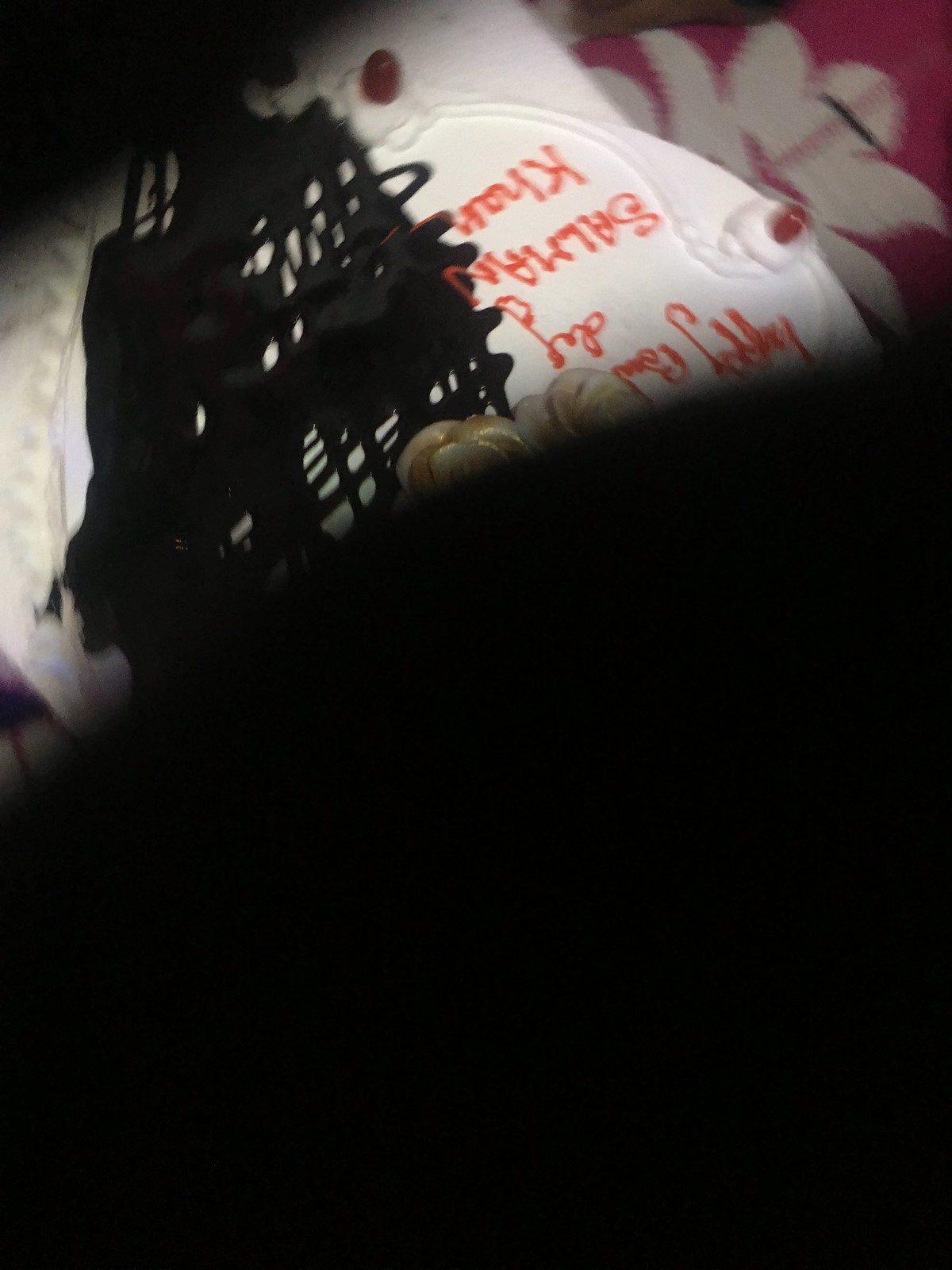An upside-down birthday cake, partially obscured by shadows, is presented against a dark background. The cake boasts smooth, white icing and features a red inscription that reads "Happy Birthday" in two distinct sections. The name "Salma Khan" is also written in red icing, although it is somewhat difficult to discern due to the shadows. The cake rests on a floral tablecloth adorned with pink and white patterns, adding a touch of elegance to the setting.